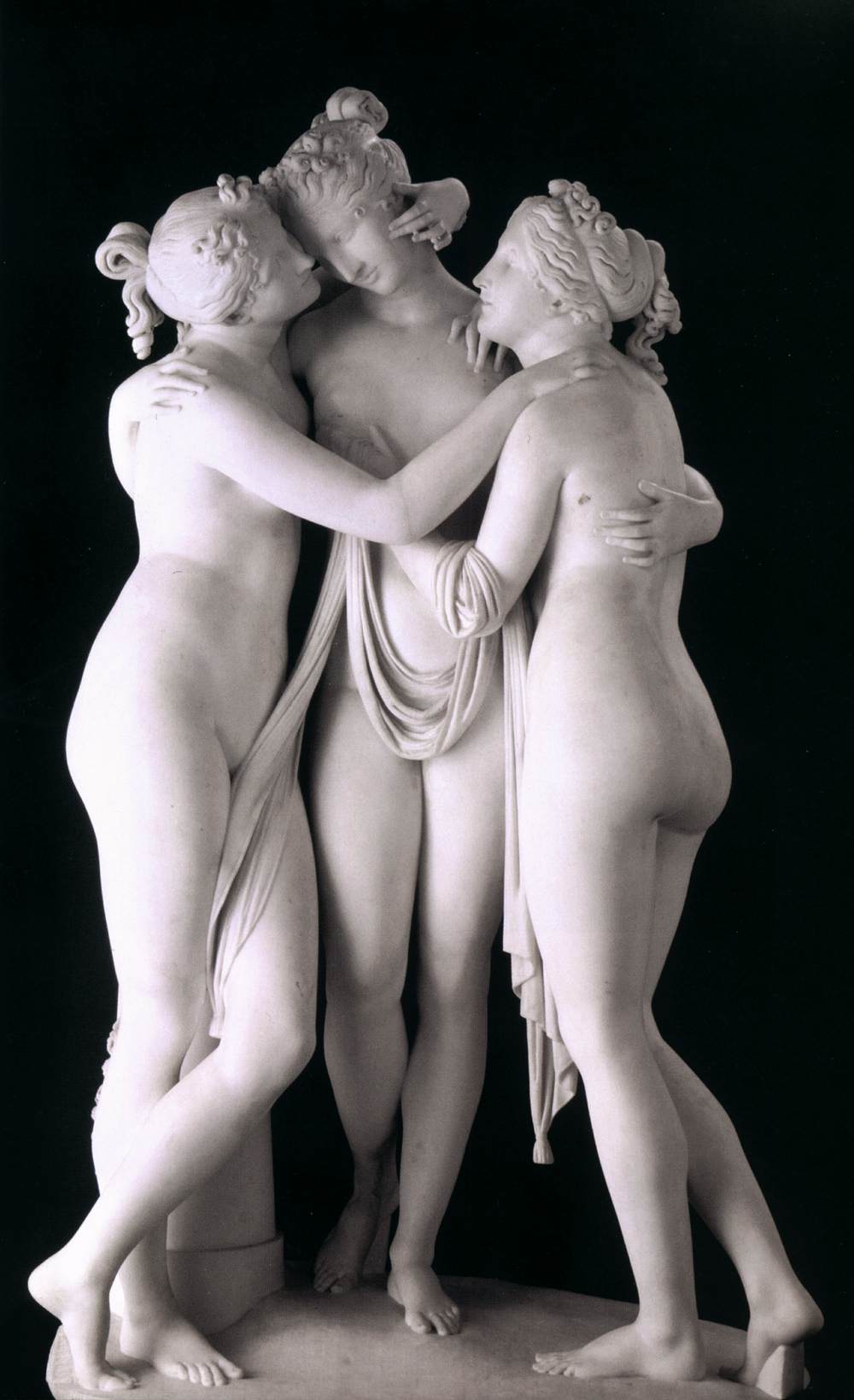This vertically aligned rectangular image features a marble statue centered against a solid black background. The statues depict three mostly naked women standing closely together, embracing one another. Each woman has her hair up in curly styles adorned with ornate headdresses. Their bodies are intertwined with mutual gestures of affection: the woman on the left is leaning into the central figure, with her arm around the latter's head and her right arm extending to the woman on the right. The central woman reciprocates by wrapping her right arm around the woman on the left and her left arm around the woman on the right. The woman on the right, partly visible from the back and side, stands with her legs crossed gracefully. A draped scarf accentuates their forms, weaving between the figures – starting from the waist of the woman on the left, looping around the middle, and over the arm of the leftmost figure. The statues stand on a partially visible circular stone base. The clean, white marble contrasts strikingly against the black background, suggesting an indoor setting, possibly a museum exhibit. The entire tableau emanates a serene, timeless quality, enhanced by the statue's smooth, unblemished surface in shades of white and gray.